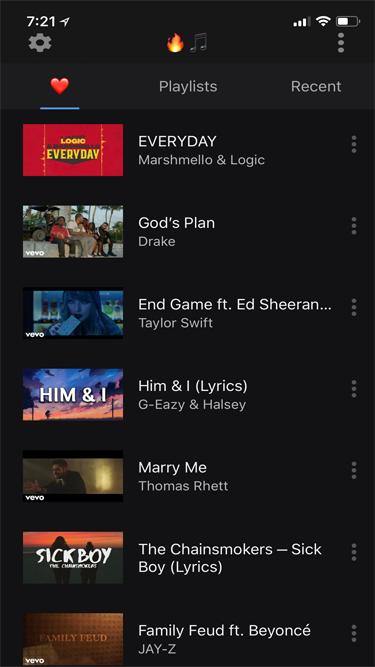This image is a screenshot from a music streaming service interface, showcasing a list of seven popular songs, each accompanied by its thumbnail on the left. At the top of the list are three navigational icons: a red heart on the left with a blue line underneath it, indicating it as the active selection; "Playlists" in the center; and "Recent" on the right.

Following the navigation icons, the list of songs starts with "Every Day" by Marshmello and Logic. Just below it is "God's Plan" by Drake, followed by "End Game" featuring Ed Sheeran by Taylor Swift. Below Taylor Swift's song is "Him & I" by G-Eazy and Halsey. Further down the list is "Marry Me" by Thomas Rhett. The sixth song is "Sick Boy" by The Chainsmokers, and the last entry is "Family Feud" featuring Beyoncé by Jay-Z. Each song entry includes its respective thumbnail on the left, and the song's name is prominently displayed next to it.